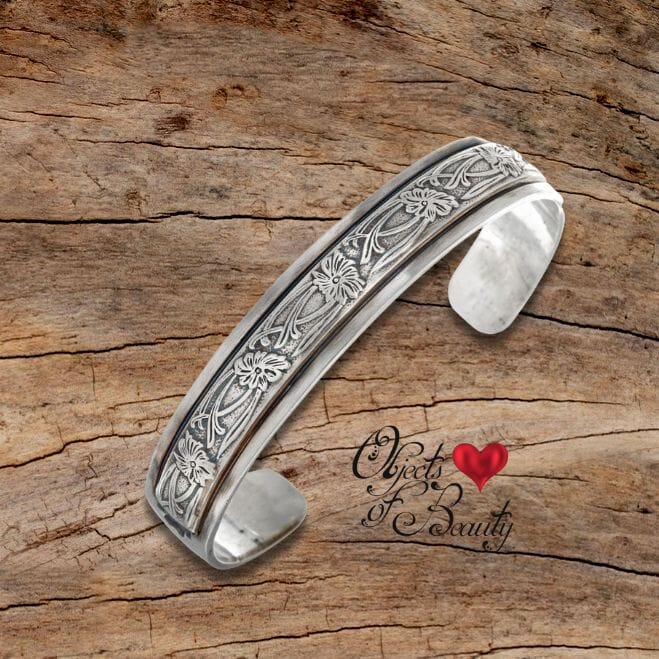The image features a silver cuff bracelet intricately engraved with a continuous pattern of flowers, leaves, and stems along the entire band. This bracelet, designed to fit various wrist sizes, prominently displays the phrase "objects of beauty" in elegant cursive just below the floral etchings, accompanied by a striking red 3D heart symbol. The bracelet is set against a rustic wooden background that appears to be a tree stump, highlighting its artisanal quality. This professionally staged product photo, likely intended for an online marketplace such as Etsy, emphasizes the craftsmanship of the bracelet and its appeal as a beautiful, handmade accessory.